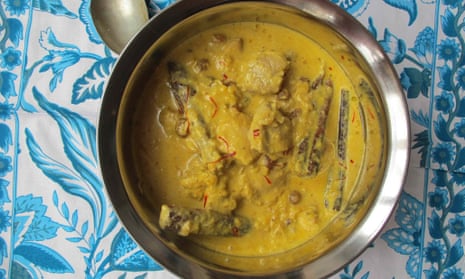A vibrant image showcases a steaming bowl of soup with a rich, yellow broth. Within the soup, a generous assortment of chunks, likely pieces of tender chicken, and a few visible bones suggest a hearty, homemade quality. Speckled throughout the broth are thin, red strips, possibly slices of red pepper, adding a splash of color and hinting at a flavorful spice. The soup is contained in a sturdy, metallic bowl, viewed from an overhead angle.

To the top left of the bowl, the rounded part of a metal spoon peeks into the frame, suggesting readiness for an impending delicious meal. The bowl and spoon rest on a visually appealing placemat, predominantly white with an intricate blue pattern. The design features an array of floral and leafy motifs, adding an elegant touch and enhancing the overall aesthetic of the dining setup.